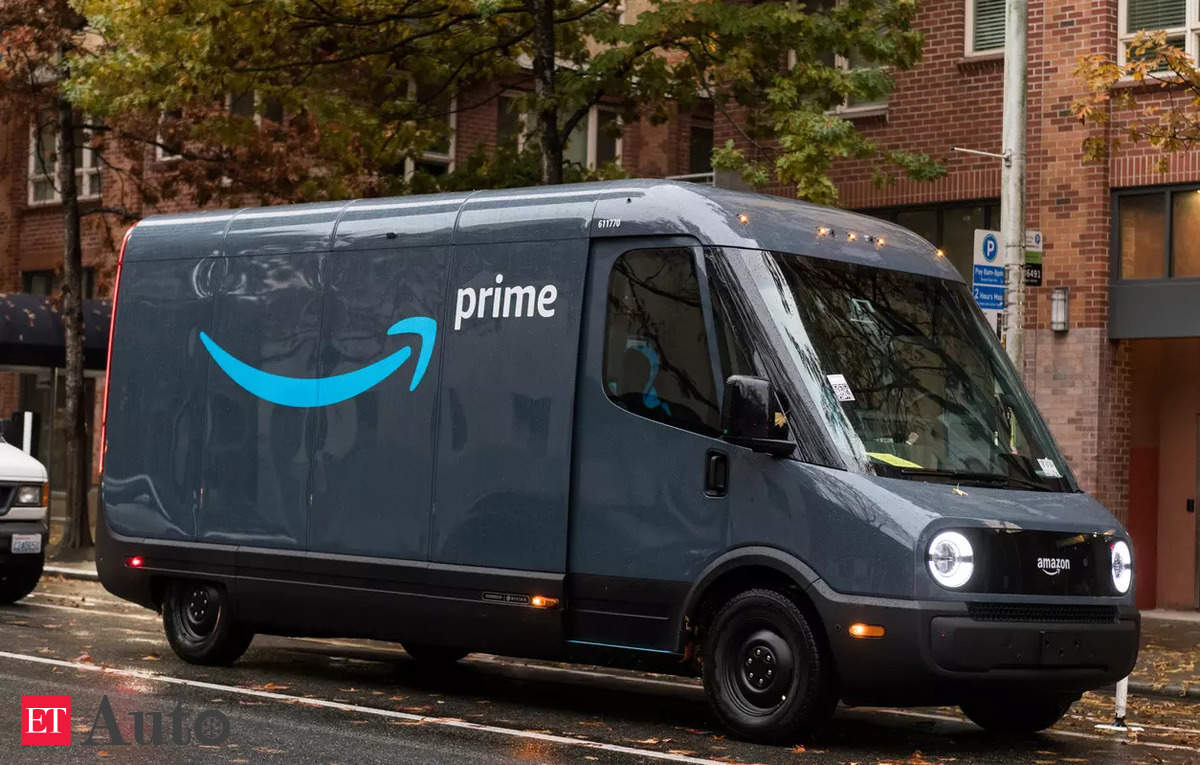The photo captures a dark blue Amazon Prime delivery truck parked on the side of a street. The truck features a prominent blue arrow on its side, accompanied by the Amazon Prime logo in white font. This delivery vehicle has a sleek design with windows only at the front, including the front windshield and doors; the back section remains windowless. 

The truck is situated next to a curb, and in the bottom left of the image, a white font reading "ET" on a red background is visible, with a gray font that says "auto" beside it. 

In the background, there is a brick building with multiple stories and numerous windows. It appears to be composed of at least two distinct sections. A few trees are positioned behind the delivery truck and in front of the brick building, adding a touch of greenery to the urban scene.